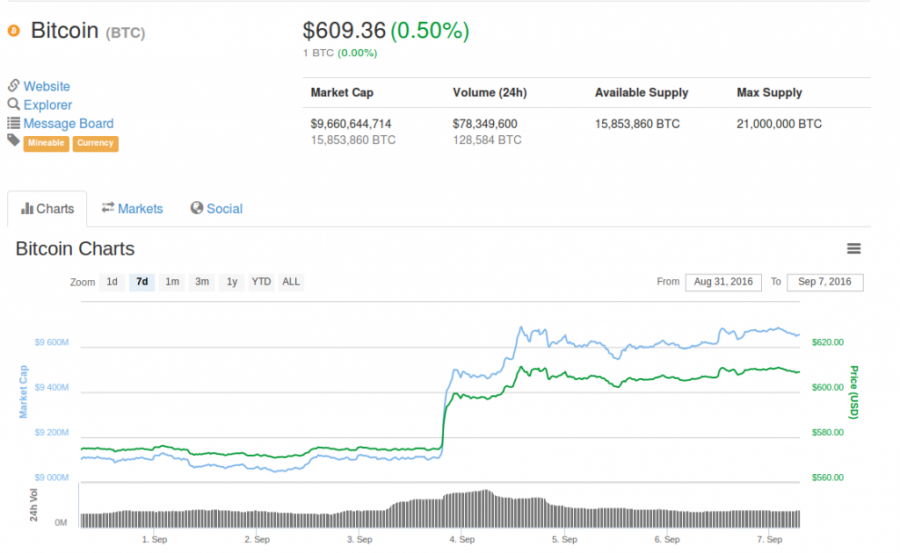The image depicts a detailed view of a Bitcoin cryptocurrency website, providing comprehensive information about Bitcoin (BTC). In the upper left-hand corner, the title "Bitcoin BTC" is prominently displayed. Adjacent to this, the current value of Bitcoin is shown as $609.36, with a percentage increase of 0.50% indicated in green.

Below this section, the website features options labeled "Website," "Explorer," and "Message Board," organized into three distinct lines in blue text for easy navigation. 

Central to the image is a chart labeled "Bitcoin Bit Charts," offering various timeframes for users to analyze Bitcoin's performance: 1 day (1D), 7 days (7D), 1 month (1M), 3 months (3M), 1 year (1Y), year-to-date (Y2D), and all-time (All). This chart visually represents Bitcoin's price trends along with its market cap fluctuations.

At the top of the chart, the market capitalization of Bitcoin is specified as $9,660,644,714, translating to 1,585,386 BTC in terms of Bitcoin units. 

Furthermore, the website provides data on the 24-hour trading volume, which is noted as $778,349,600. For clarity, the maximum supply of Bitcoin is indicated at 21 million BTC.

Overall, the image offers a thorough snapshot of Bitcoin's financial metrics and user interface on the website.